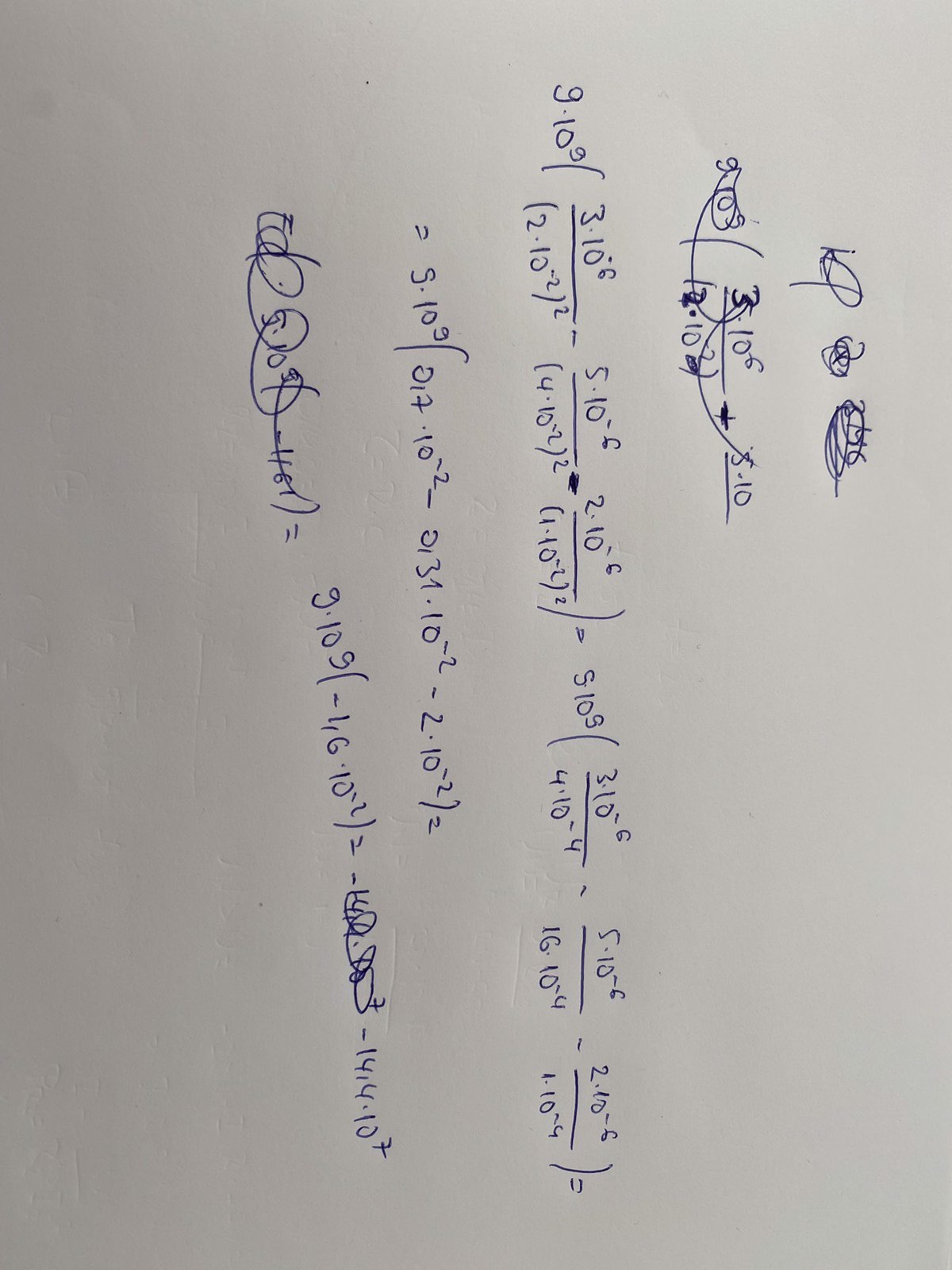This photograph captures a piece of handwritten math work oriented sideways, requiring the viewer to turn their head to the right to read it properly. The work is penned in blue ink on what appears to be standard white or gray paper. The page is densely populated with exponential equations, including a prominently written "9 x 10^9." The mathematical notations are interspersed with longer, more complex equations nested within parentheses, some of which overlap. Notably, both the top and bottom sections of the page feature scratched-out components. Above these scribbles lies a short, incomprehensible text segment, also crossed out. The detailed, overlapping, and sometimes obliterated equations suggest intense problem-solving efforts and corrections.